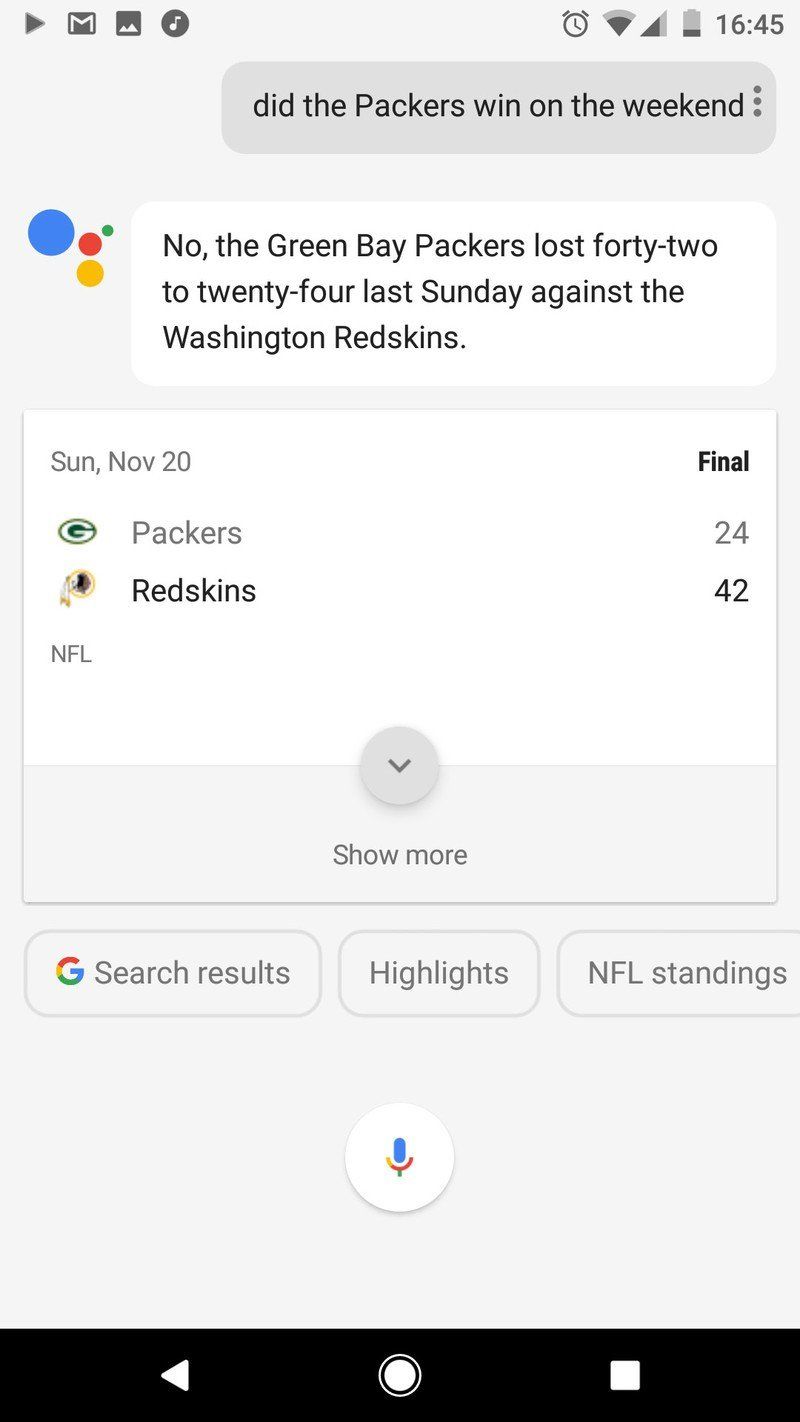The image depicts a screenshot of a mobile phone screen with dimensions approximately two and a half times taller than it is wide. In the top left corner, various app icons are visible, including the recognizable Play button and Gmail icon, along with two other indistinct icons. On the top right, there are icons representing an alarm, cellular and Wi-Fi signal strengths (both nearly three-quarters full), and a nearly depleted battery. The time displayed is 16:45.

The main content of the screen appears to be a chat interface. A gray text bubble contains black text asking, "Did the Packers win on the weekend?" The respondent's profile picture features four circles in different colors: blue, red, yellow, and green. To the right of this profile picture, a white text bubble with black text states, "No, the Green Bay Packers lost 42 to 24 last Sunday against the Washington Redskins." Below this exchange, there is a summary displaying the final score of the Packers versus Redskins game, verifying the chat message. An expandable section marked by a down arrow and labeled "Show more" is situated below the score.

At the bottom of the screen, three interactive buttons are present: one for Google search results, another for highlights, and a third for NFL standings.